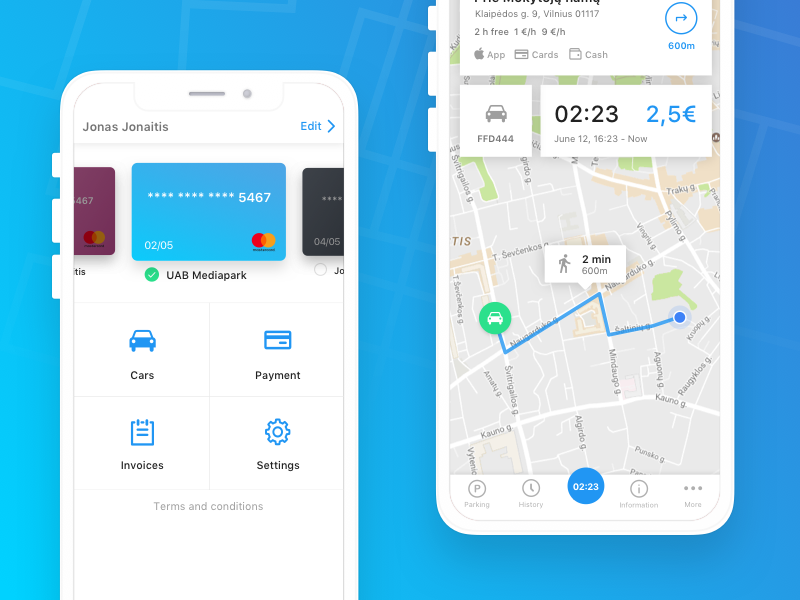The image depicts two smartphone screens side by side. The screen on the right shows a navigation map displaying a route with street names and a designated destination. Both walking and car icons are visible, indicating different travel mode options. The estimated travel time is 2 minutes and 23 seconds, and the cost is displayed as 2.5 euros. 

The screen on the left shows a digital interface where the user can select a payment method. A credit card is prominently displayed, suggesting that this is the chosen payment option. Below the credit card, there are tabs labeled "Cars," "Payment," "Invoices," and "Settings," indicating different sections of the application. The overall context suggests that the user is setting up payment for a short trip using a ride-sharing service.